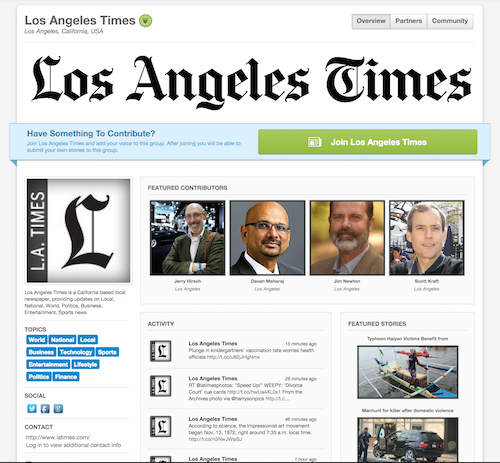This image is a detailed screenshot of the Los Angeles Times website. The edges of the website are flanked by white-gray sidebars, framing the primary content area, which is set against a white background. 

At the very top of the page, the header prominently displays "Los Angeles Times," accompanied by a green circle featuring a downward arrow. Directly below this, the text "Los Angeles, California, USA" is displayed. 

To the right of the header, there are navigation links labeled "Overview," "Partners," and "Community."

Just beneath the main header, "Los Angeles Times" is repeated, followed by a striking blue banner. This banner calls for engagement, inviting users to "Have something to contribute?" in bold blue print. Below this message, the banner encourages visitors to "Join Los Angeles Times and add your voice to this group," explaining that as members, users can submit their own stories. The call-to-action is reinforced by a prominent green button that reads "Join Los Angeles Times."

Further down the page, more navigation options are available, including links to "Featured Contributors" and "Activity." A comprehensive list of news categories is also visible, covering diverse topics such as World, National, Local, Business, Technology, Sports, Entertainment, Lifestyle, Politics, and Finance. 

Additionally, there is an option labeled "Show Social Contact," suggesting social media integration or contact options. 

On the right-hand side of the page, several featured stories are displayed with accompanying images, although the lower parts of these images appear to be cut off in the screenshot.